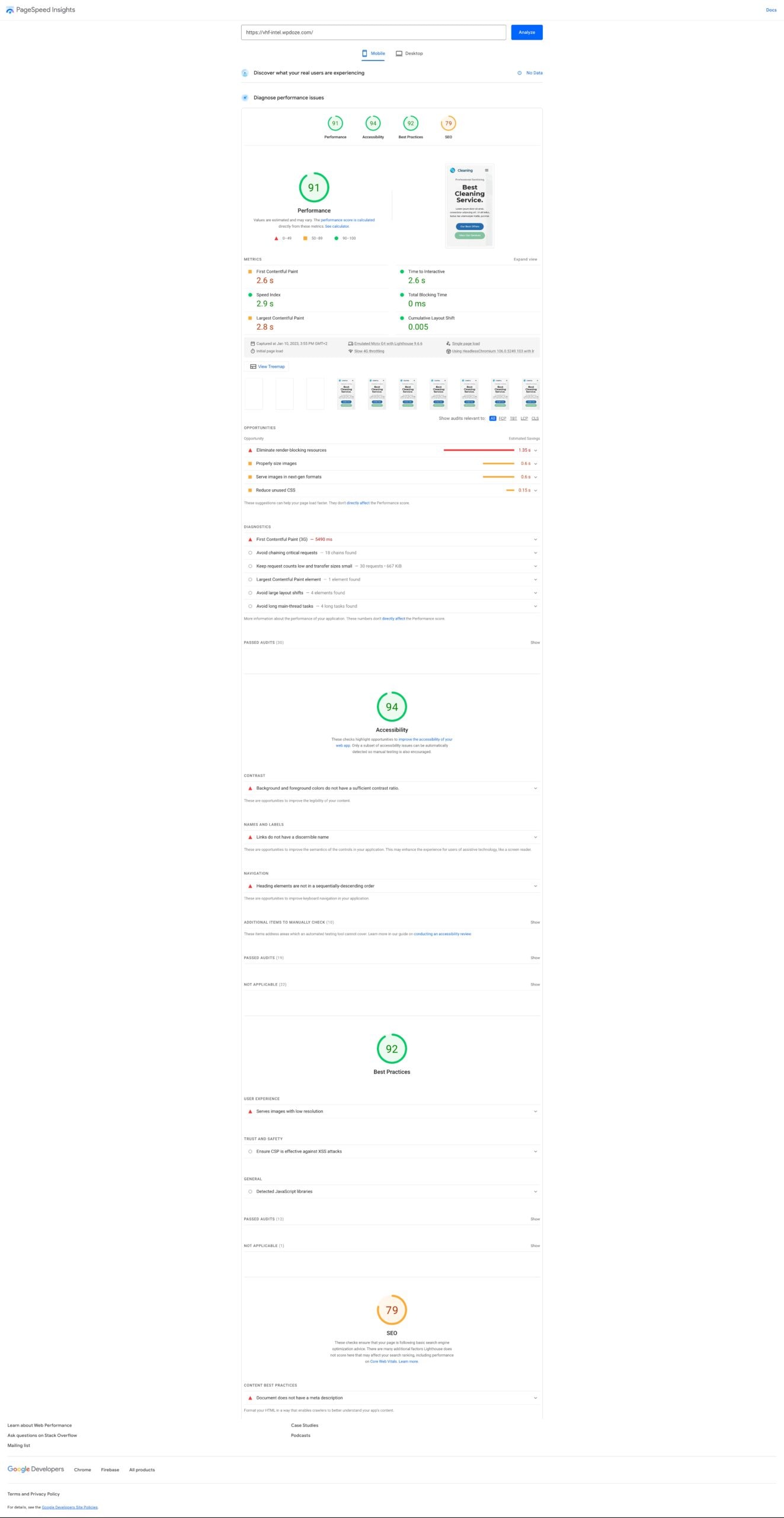A small screenshot of a website with a white background dominated by multiple circular graphs, unable to be viewed clearly due to the image’s diminutive size. At the top of the page, five circular graphs are visible, four of which are green and one yellow. Each graph prominently displays a numerical percentage in its center, likely indicating some form of data metric. The font across the website is black, though the text descriptions accompanying the graphs are tiny and unreadable. Additional circular graphs appear as you scroll down the page, with two green circles labeled 91% and 92%, respectively, and another yellow circle at the bottom showing 79%. The content of the website seems lengthy, filled with numerous detailed descriptions accompanying these graphical representations.